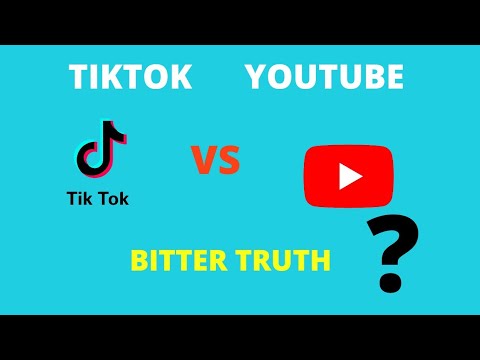This rectangular image, with a slightly longer horizontal dimension, features distinct sections and vibrant color contrasts. The top and bottom sections are bordered by black strips, framing a central turquoise field. At the top left, "TIKTOK" is displayed in uppercase white text, mirrored on the right by "YOUTUBE," also in uppercase white text. 

Central to the composition, the TikTok logo—a distinctive black and pink musical note—sits prominently above the word "TikTok," which is written in a mix of capital and lowercase black letters. Below this, "VS" is boldly printed in red, flanked by the YouTube logo, which is depicted as a red rectangle containing a white play button. Directly below this, the phrase "BITTER TRUTH" is written in all caps with a yellow font. 

A large, solid black question mark, about two and a half times the size of the surrounding text, adds a bold, inquisitive element near the bottom. However, the YouTube icon appears slightly misaligned, nearly touching the oversized question mark, which in turn seems disconnected from the "BITTER TRUTH" text due to excessive spacing. This arrangement and spacing issue slightly detracts from the overall cohesiveness and clarity of the design, suggesting the image's intent to compare TikTok and YouTube under the theme of "Bitter Truth."